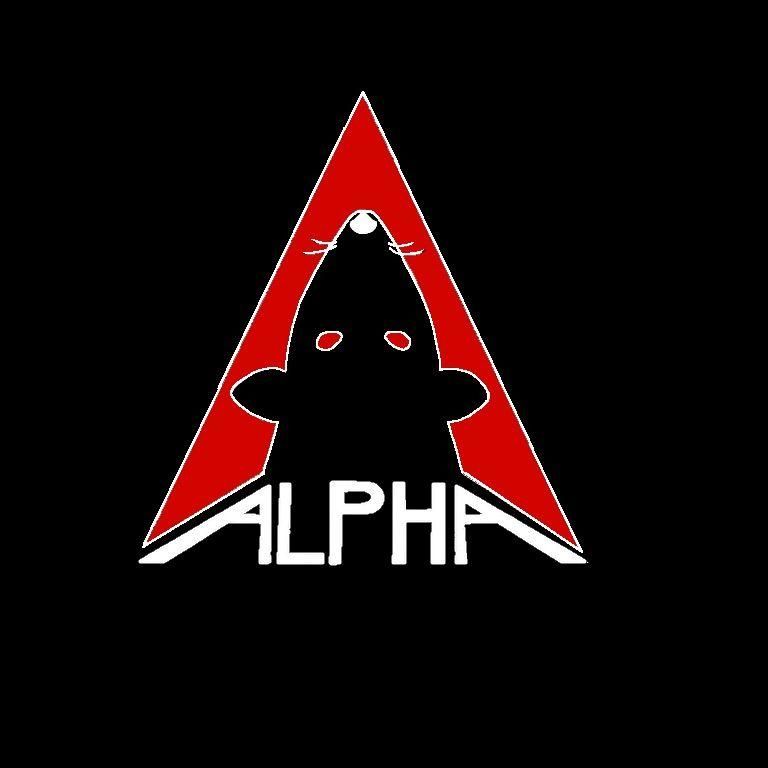In the center of the image against a pure black background, a sleek black mouse with a prominent white nose and four distinct white whiskers gazes upward. Its ears are clearly visible, and its eyes appear red, blending with the surrounding elements. This mouse is set in the middle of a vibrant red triangle, which is sharply outlined in white. Below the mouse, fitting perfectly along the base of the triangle, is the word "ALPHA" in all capital white letters. The first and last 'A's extend diagonally outward to the left and right respectively, enhancing the futuristic and dynamic feel of the image. The entire composition exudes a modern, science-fiction aesthetic.